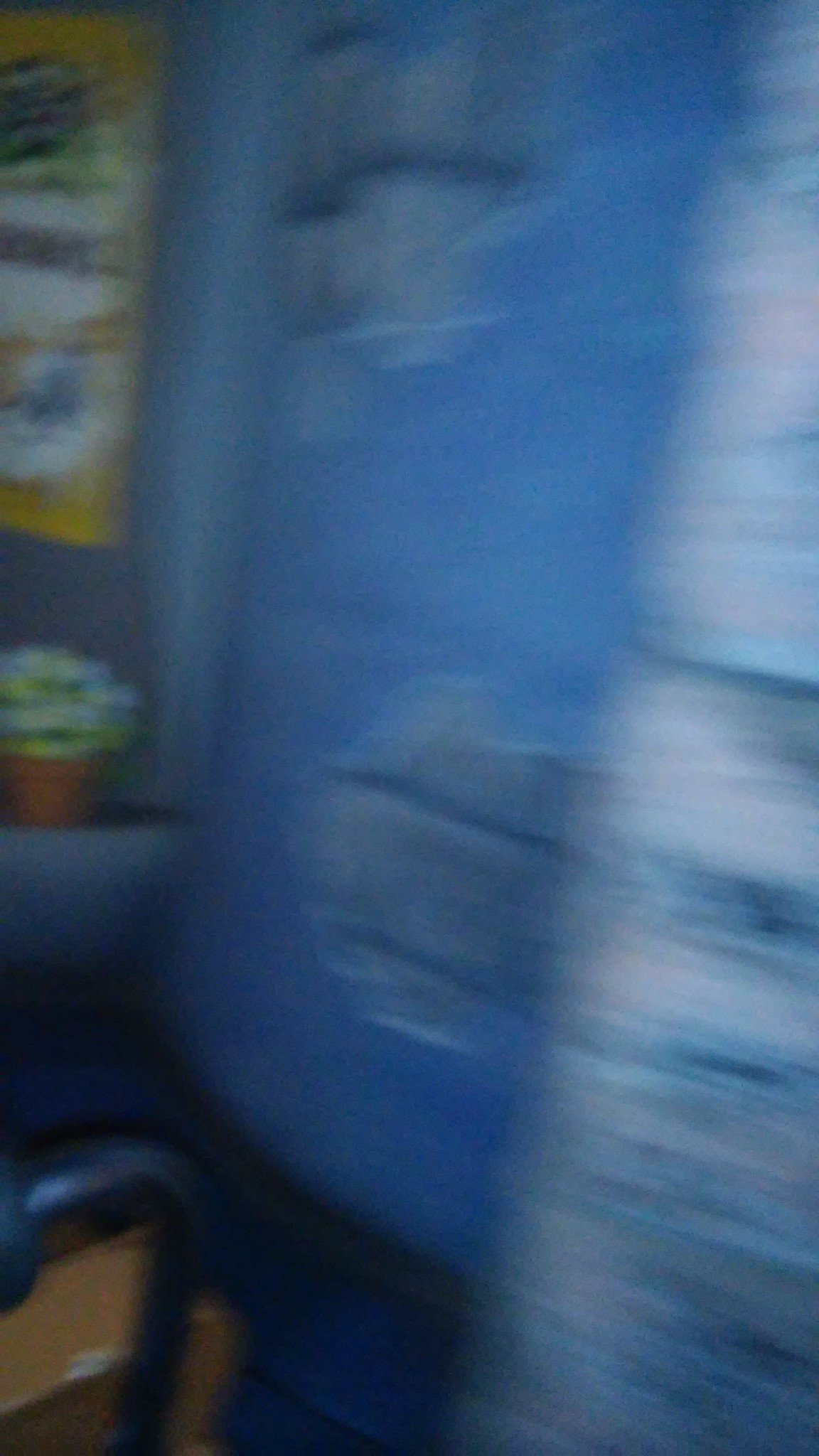This extremely blurry photograph, taken in portrait mode, primarily features a large, indistinct blue rectangle at the center, possibly the back of a well-worn seat. The predominant color is blue, with potential signs of wear and threadbare patches. To the right, there appears to be a stacked white object with a hint of blue. In the upper left corner, there is a very blurred yellow poster on the wall, possibly with some blue and white details. Below the poster, a green potted plant with white and yellow flowers is faintly visible in a terracotta pot. The lower left-hand corner shows a brown object, likely a cardboard box, and a curved metal handle, which may belong to a dolly or chair. The overall scene is difficult to discern due to the extreme blurriness, adding to the ambiguity of the objects present.